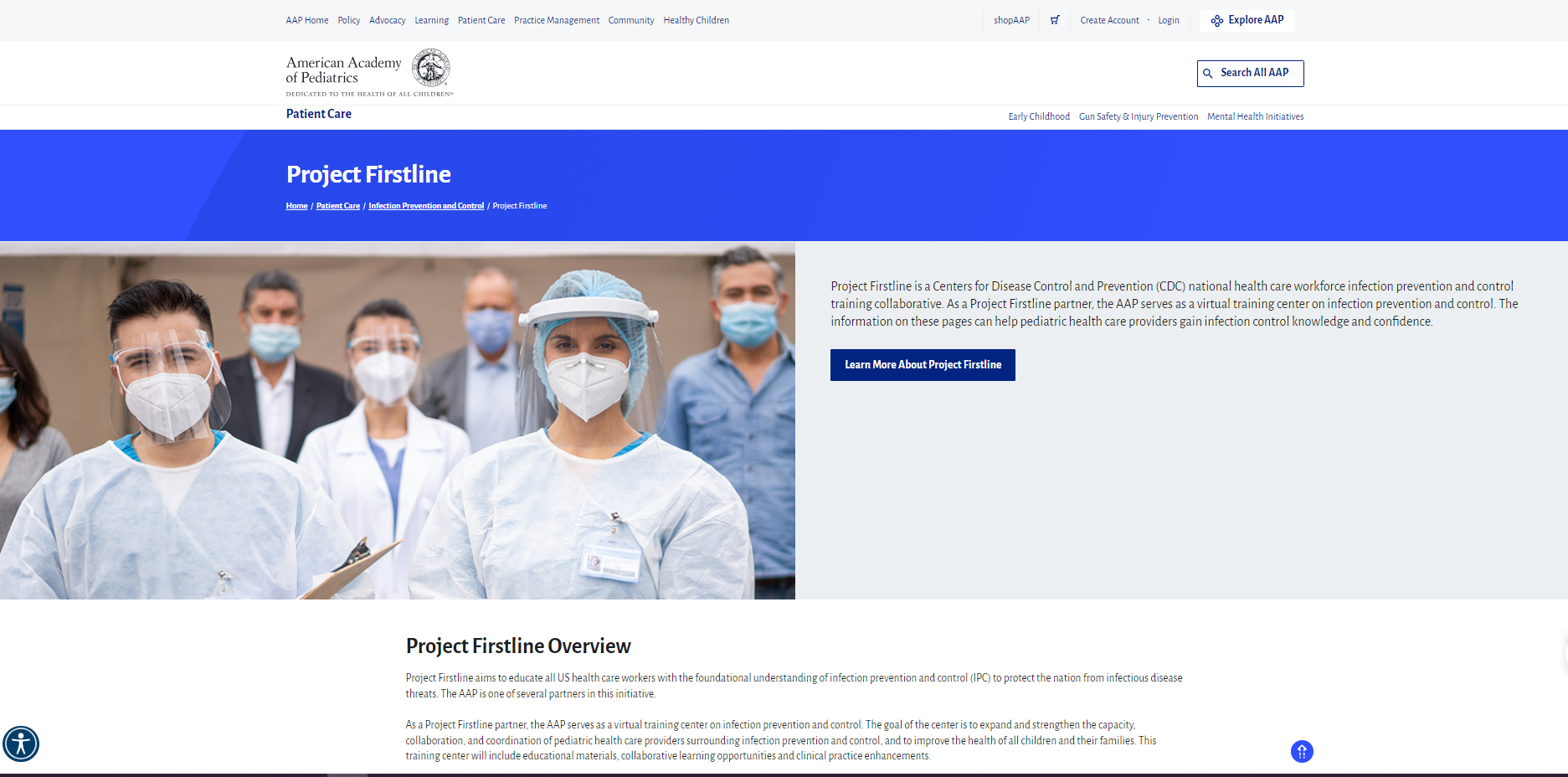**Screenshot Description: American Academy of Pediatrics Website**

The screenshot is from the American Academy of Pediatrics (AAP) website. At the top 10% of the page, there is a gray horizontal navigation bar with clickable blue text options. Towards the top right of this bar, there is a white rectangle containing the text "Explore AAP" accompanied by a logo. Directly beneath this white button, there is a blue outlined, white-filled box with the text "search all AAP".

On the left side of the gray bar, the words "American Academy of Pediatrics" are displayed in black text. Below this, the phrase "Patient Care" is featured in blue text.

Spanning across the screen below the navigation bar is a fairly large horizontal blue rectangle with white text that reads "Project FirstLine". Underneath this blue rectangle, there is an image depicting several doctors all wearing white masks. Most of the doctors are dressed in white gowns, except for a few individuals in the background: one woman is wearing gray, a man is in dark gray, another man is in light gray, and one more man is wearing blue attire. 

To the right of the image, there is a dark blue button that reads "Learn more about Project FirstLine".